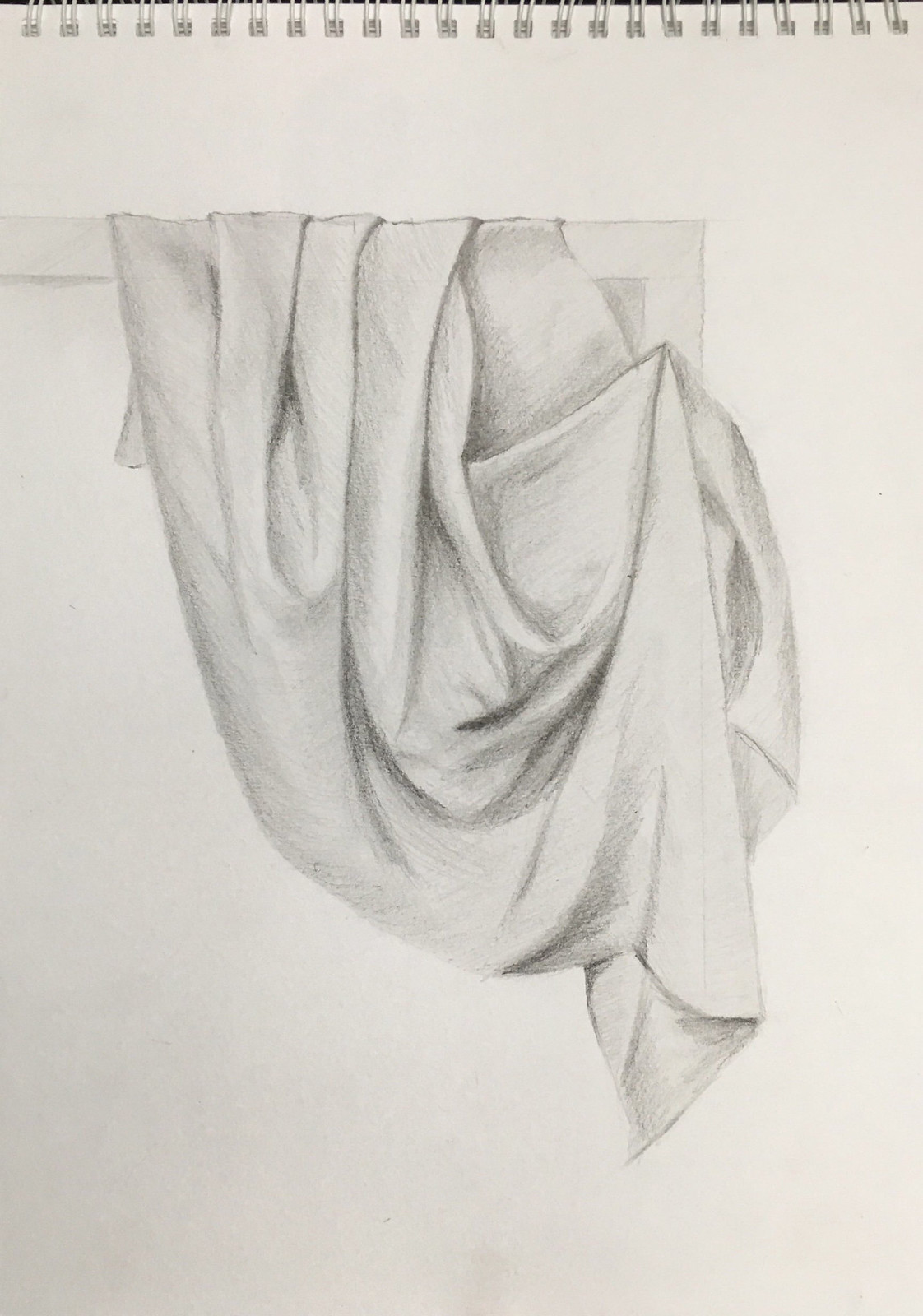This detailed black-and-white pencil drawing depicts a piece of cloth intricately draped and folded over an unspecified wooden structure, possibly a window frame. The cloth, rendered with meticulous shading, forms a cradle-like shape at its center, adding depth and dimension to the image. The folds are pronounced and contribute to the realistic texture of the fabric, showcasing the artist's skill in capturing the delicate interplay of light and shadow on a simple white background. The composition emphasizes the elegance and simplicity of the draped cloth, drawing attention to its elaborate and carefully crafted design.